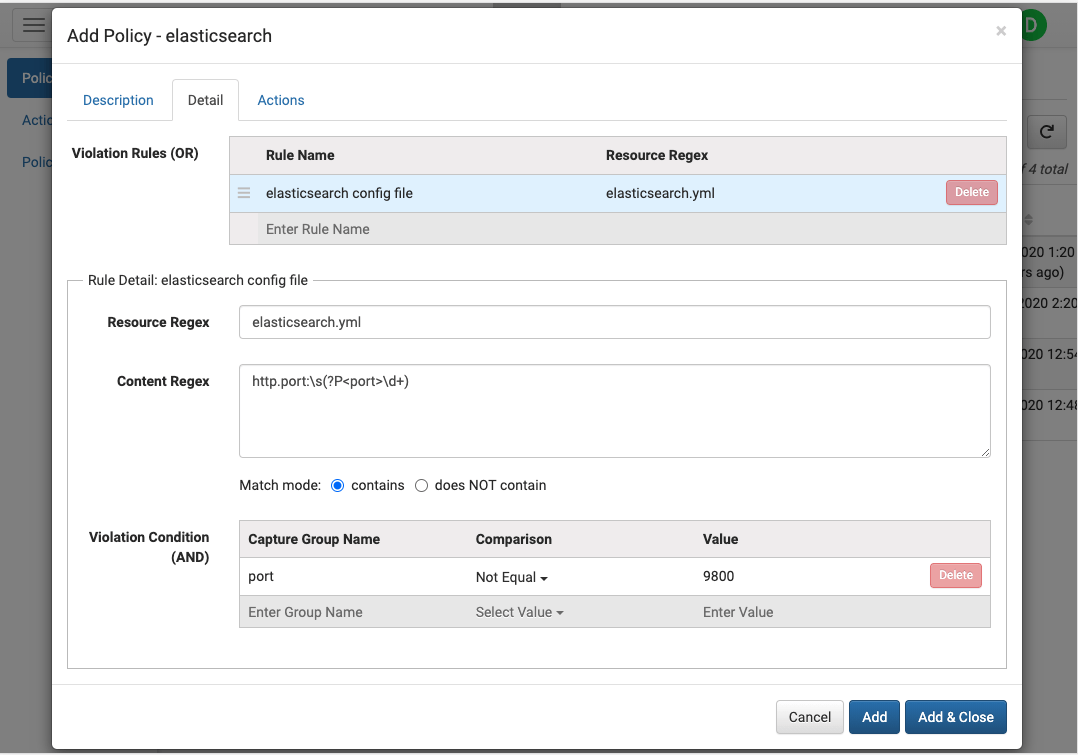In this image, a pop-up titled "Add Policy: Elastic Search" is prominently displayed at the top left in bold black text. Directly below the title are three interactive tabs labeled "Description," "Detail," and "Actions" from left to right. The middle tab, "Detail," is currently selected, indicated by its black color, while the other tabs are blue.

The section below the tabs is titled "Violation Rules." Here, a rule named "Elastic Search Config File" is listed. The resource associated with this rule is designated by the regex "Elastic Search YML". 

Further down, there are forms for entering details: "Enter Rule Name" and "Rule Detail," which includes fields for specifying the "Elastic Search Config File," "Resource REGX," and "Content REGX." An additional option below this is labeled "Match Mode," offering a choice between "Contains" and "Does Not Contain" with the former selected, highlighted by a blue circle around the word "Contains."

The next section is titled "Violation Condition," which features three categories for input: "Capture Group Name," "Comparison," and "Value." Within this section, it specifies "Port," "Not Equal," and "9800" respectively. There is also a "Delete" button located to the right of these inputs. 

Under the violation conditions, there are prompts for entering more data: "Enter Group Name," "Select Value," and "Enter Value."

At the bottom of the pop-up are three buttons arranged from left to right: a silver "Cancel" button, a blue "Add" button, and another blue button on the far right labeled "Add and Close."

Flanking the pop-up on both sides is a light gray background extending from top to bottom.